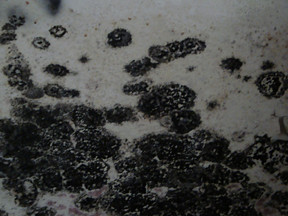This black and white, rectangular image, captured through a microscope, showcases what appears to be a close-up of cell culture or possibly an infestation of organic mold or fungus on an off-white background. The photograph reveals several circular or near-circular black shapes, some clustered in groups while others are isolated. These shapes look organic, possibly mold or spores, exhibiting a blooming pattern against the white backdrop. 

Notably, the top and right sections of the image show a clearer view of the off-white background with sparse speckles of darker colors. In contrast, the bottom right and far left areas are densely populated with these black shapes, almost to the point of becoming solid black. This crowded clustering suggests a spreading effect, where the shapes lose their defined circular forms and merge into larger dark patches. The overall impression is somewhat unsettling, evoking the appearance of an invasive organic growth proliferating across a surface.